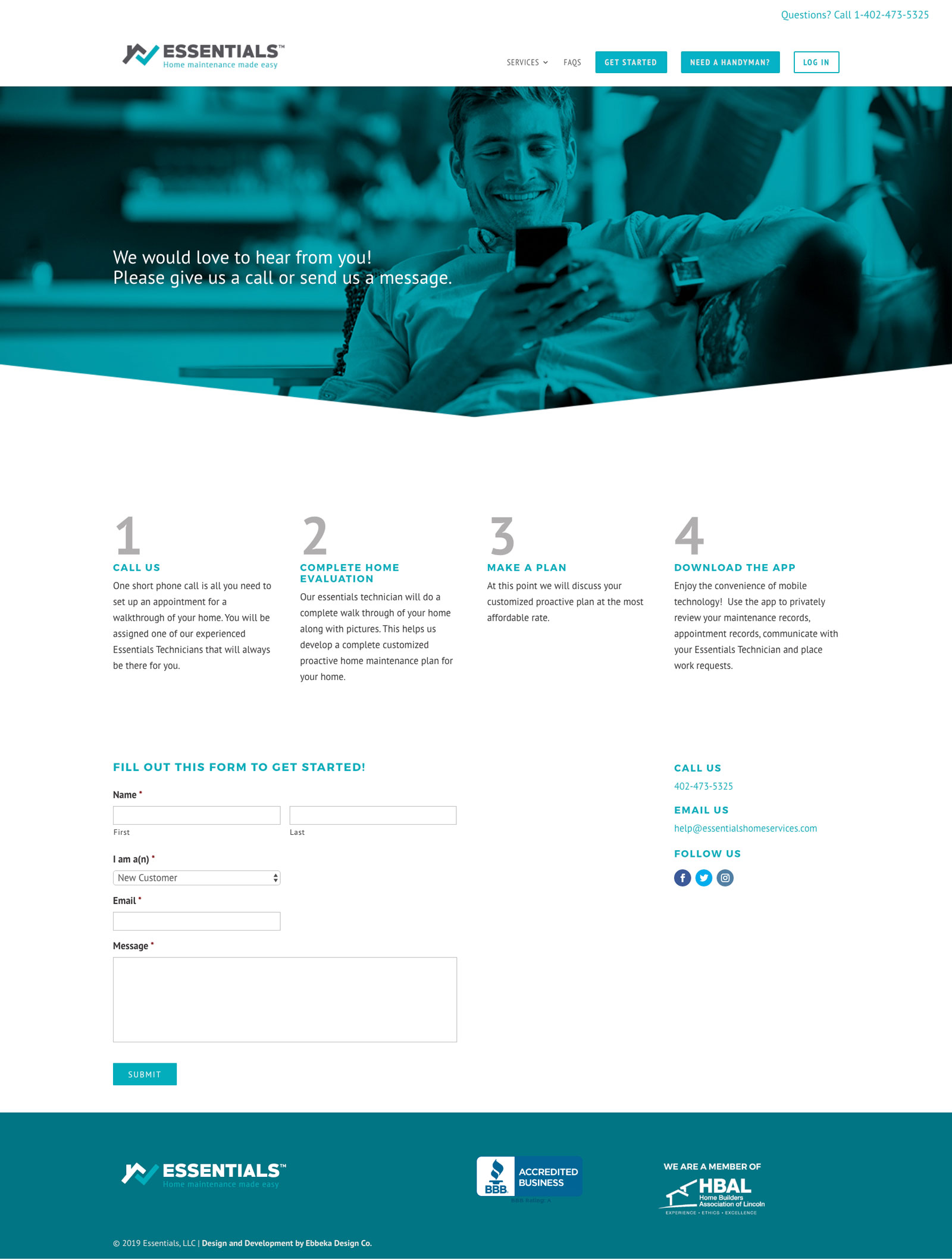The image features a detailed layout, segmented into various components:

- **Top Section**:
  - **Background**: White.
  - **Left Side**: A gray house roof icon above a check mark resembling a tail in design. Below this, in gray text, it says, "Essentials," and in teal, "Home Maintenance Made Easy."
  - **Right Side**: In teal, the word "Questions?" followed by a teal question mark icon and the phone number "1-402-473-5323." Below this, in gray, it says, "Services Frequently Asked Questions."

- **Middle Section**:
  - Two teal boxes with white backgrounds. The first box reads, "Get Started," and the second one reads, "Need a Handyman?" 
  - Another box has a white interior with a teal outline border, containing the word "Login" in teal.

- **Main Image**:
  - A man is sitting or reclining on a chair or couch. He is wearing a button-down shirt and a watch, smiling as he looks at a black electronic device. The background has a teal filter.
  - To the left of this image, in white text, it says, "We would love to hear from you! Please give us a call or send us a message."

- **Numbered Steps**:
  - Gray numeral "1" and teal text, "Call Us."
  - Gray numeral "2" and teal text, "Complete Home Evaluation."
  - Gray numeral "3" and teal text, "Make a Plan."
  - Gray numeral "4" and teal text, "Download the App."
  - Beneath these steps, in teal text, it says, "Fill out this form to get started."

- **Form Section**:
  - The form includes fields for "Name" with a red asterisk, "First Name," "Last Name," "I am a" dropdown with "new customer" as an option, "Email" with a red asterisk, and "Message" with a red asterisk.
  - At the bottom, a teal button labeled "Submit."